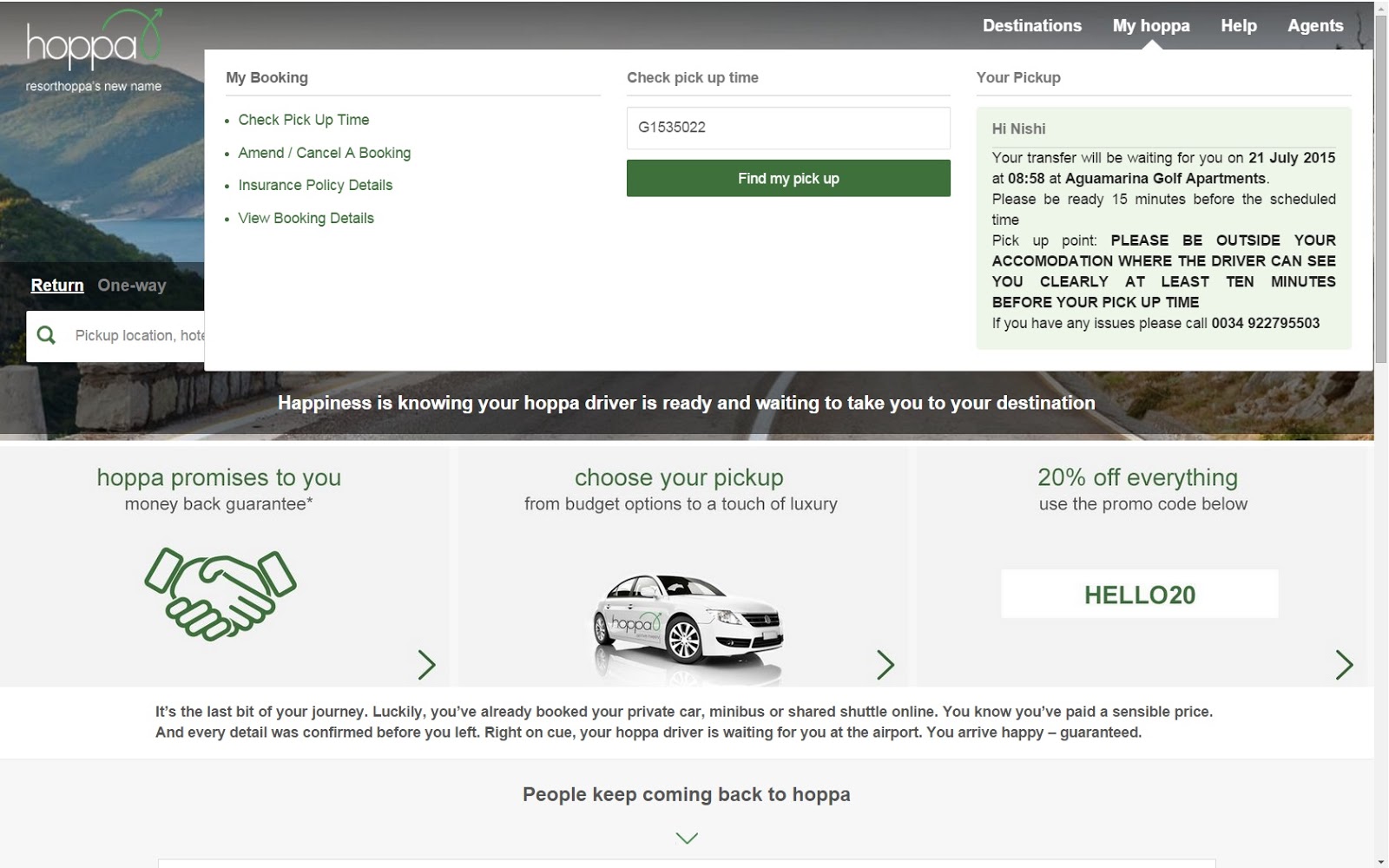The image displays a webpage for "Resort Hopper," with the name prominently shown in the top-left corner. The header features several navigation links including "Destinations," "MyHopper," "Help," and "Agents." Below these, there are additional links such as "My Booking," "Check Pick-Up Time," and "Amend/Cancel a Booking." The page offers various service details, advertising options for selecting a pick-up service ranging from budget-friendly to luxurious choices. A highlighted promotion offers 20% off all services with the use of promo code "HELLO20." The page also emphasizes a "Money-Back Guarantee" as a commitment from Hopper to assure customer satisfaction.